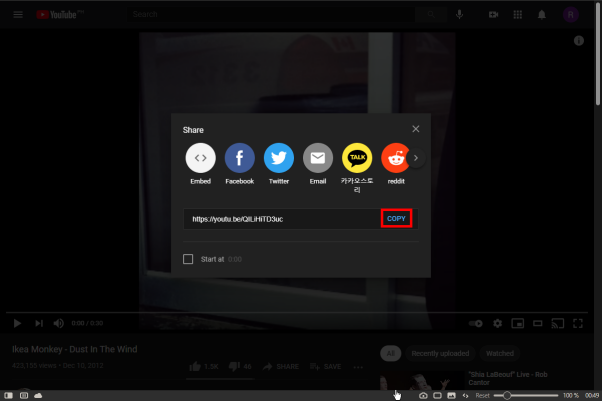A detailed screenshot from a YouTube webpage displayed on a laptop screen. The user has searched for "IKEA Monkey Duet in the World" or "Dust in the Wind," suggesting a song performance. The search results show the video page, with the user having clicked on the video to start playing it, indicated by the video starting at 00:00. The user has then selected the share button, prompting a pop-up window to appear. This pop-up window, which greys out the rest of the screen, provides several sharing options, including buttons for embedding the video, sharing via Facebook, Twitter, email, another messaging app, and Reddit. Below these options, there is a visible URL of the YouTube video and a "copy" button. This "copy" button is distinctively highlighted by a red box that appears to be digitally added to draw attention, likely encouraging the user to copy the video link. This edited emphasis suggests that the user plans to copy the URL for sharing, either via email or through another messaging service.